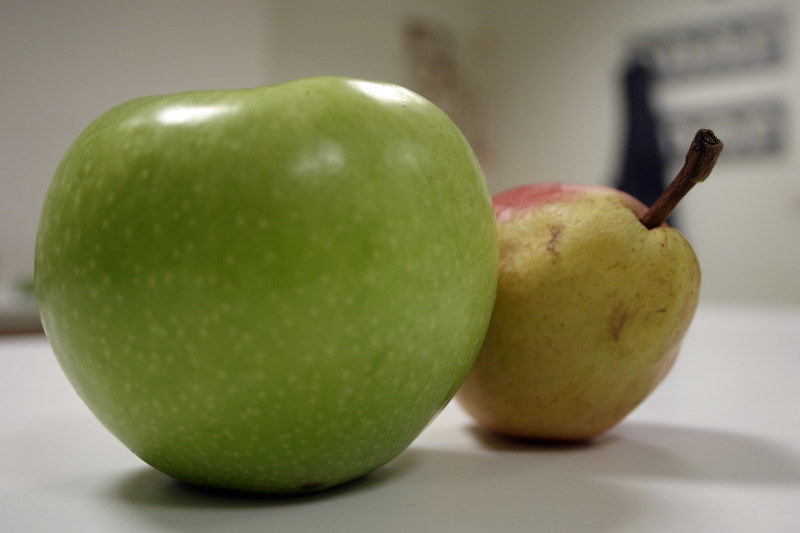The image showcases two pieces of fruit placed side by side on a pristine white countertop. On the left, there is a large, vibrant green apple, reminiscent of a Granny Smith variety, freckled with a few natural spots and lacking a stem. To its right stands an elegantly multicolored pear, featuring a harmonious blend of reddish and brownish hues that gently transition into a greenish-beige area, all crowned with a distinct long brown stem. The fruits appear fresh and enticing, particularly the lush green apple. In the blurred background, two decorative signs are barely discernible, adding a subtle touch of depth to the otherwise simple and colorful composition. The image captures the natural allure of the fruits in a minimalistic yet engaging manner.